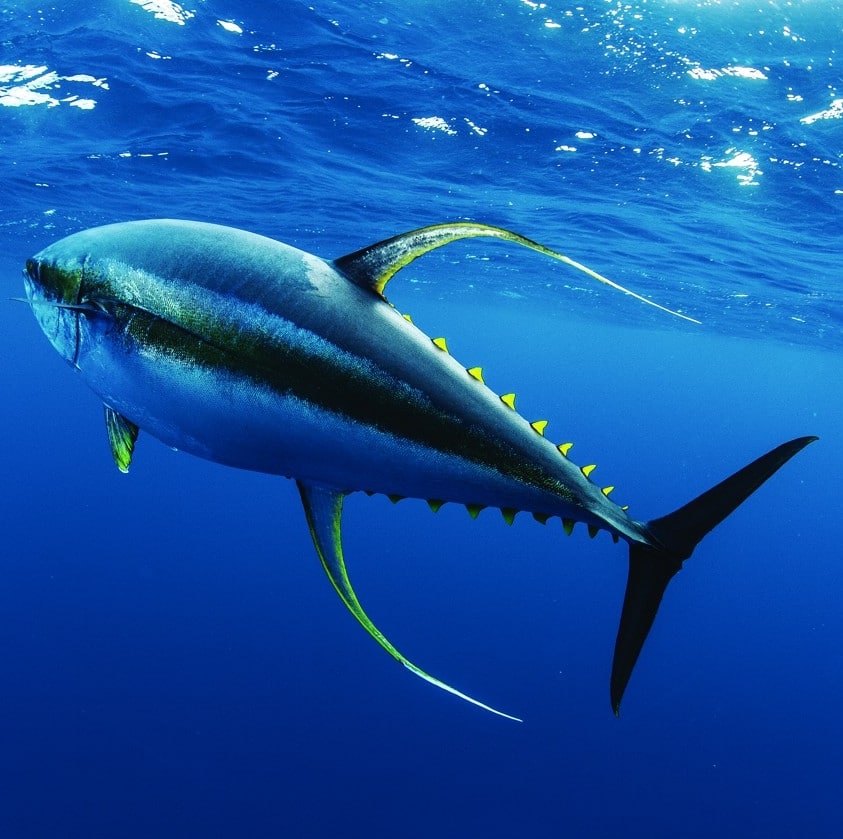This image captures a vividly blue-hued yellowfin tuna gliding just beneath the clear ocean surface, pointed to the left. The backdrop is predominantly bright blue, with solid blue at the bottom and wave patterns at the top, indicating the water's surface. The tuna is distinguished by a black stripe running along its side, yellow fins on its tail and sides, and particularly notable sharp, yellow fins along its back. Its sleek body shows a harmonious blend of blue and yellow tones, exhibiting nine pronounced dorsal fins and two long side fins with a thin yellow stripe. The overall scene is serene, providing a detailed look at the yellowfin tuna's graceful, solitary swim in its natural habitat.